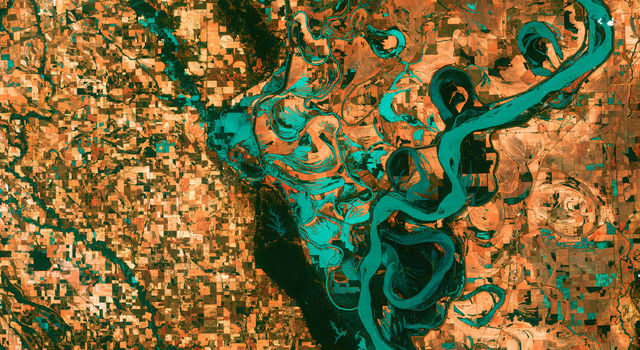An aerial image showcasing a vividly colored geographical landscape. The primary hues are yellow and blue, creating a visually striking contrast. The scene includes a central area of bluish-green water with swirling patterns, reminiscent of an abstract painting. Surrounding this water body are various dark, square-like patches scattered across the predominantly yellow terrain, adding texture to the composition. The intricate interplay of colors and shapes suggests a detailed map or an artistic interpretation of a landscape from an overhead perspective.